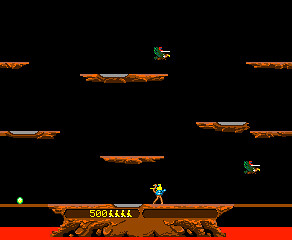This screen capture from what appears to be a retro video game showcases a black background with a distinctive pixelated design. The upper two-thirds of the screen features approximately five to seven evenly spaced horizontal floating platforms, colored in orange. Just right of center in the upper portion, there is a green character with a hint of red, likely a dragon or another fantastical creature, which might also carry a person on its back. The lower portion of the image displays a ground section composed of a brown plateau or rock outcrop emerging from a vibrant red stripe, likely indicating lava. Near the center and slightly to the right, another character is visible, an ostrich-like creature with long legs and blue feathers, also seemingly ridden by a person dressed in yellow. Alongside this character, the rock outcrop is marked with a digital score of '500' and four additional yellow symbols. To the far left on the ground level, a green dot or object can be seen, adding to the complex visual scene.